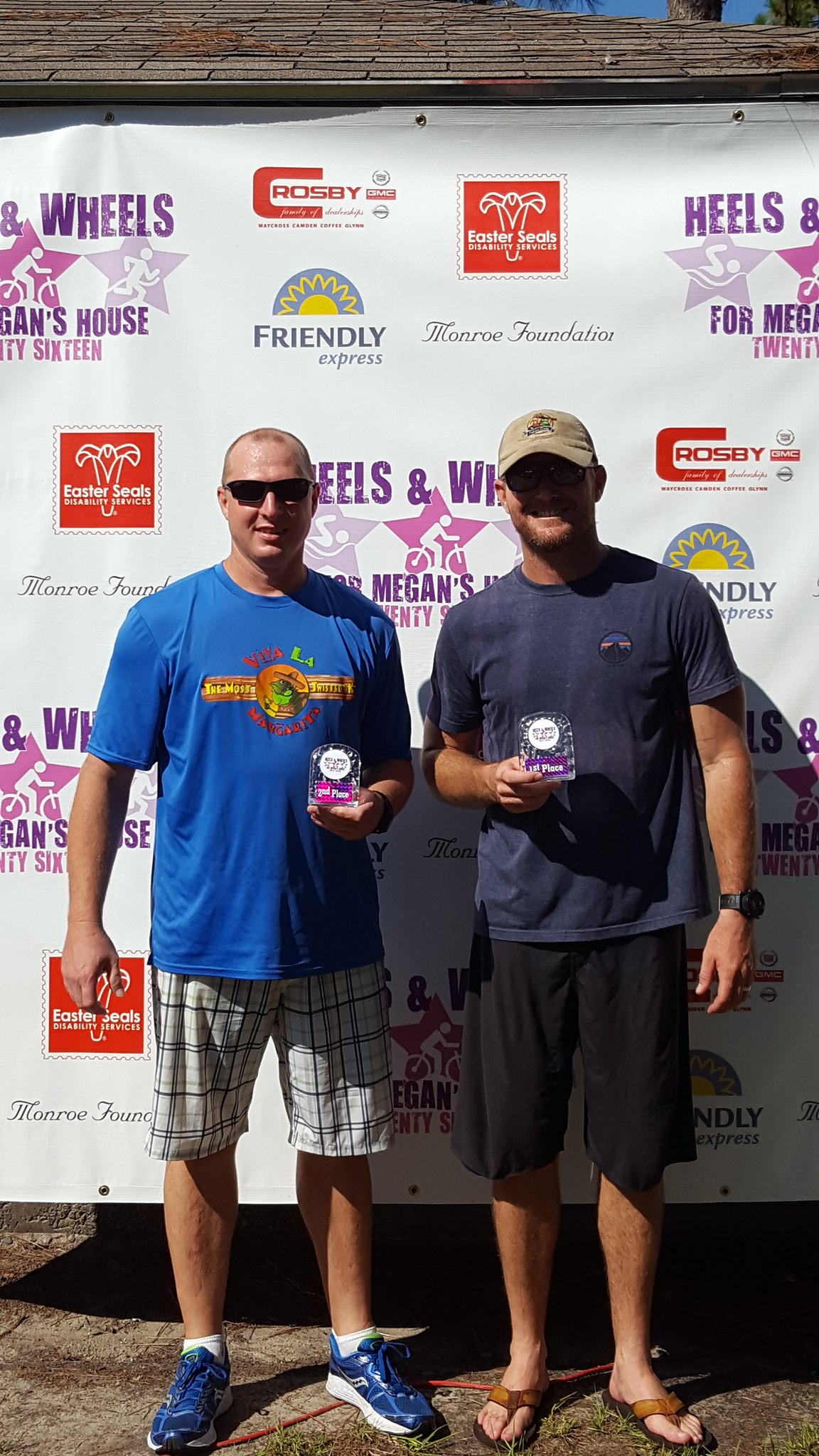Two men stand in front of a large white banner adorned with various logos and text. The banner, which spans from a wooden top rail down to just above the men's feet, prominently features logos for "Easter Seals Disability Service," "Heels and Wheels for Megan's House 2016," "Friendly Express," and "The Monroe Foundation." Both men, who are white and wearing shorts, are holding small crystalline trophies.

The man on the left is bald and wearing sunglasses, a blue T-shirt with red and green text, possibly reading "Viva La Margarita" with a frog logo, plaid light blue and white shorts, and bright blue sneakers. He is holding a pink trophy in his left hand that reads "Second Place." The man on the right has a beard and is wearing a beige-colored hat, a dark blue T-shirt, black shorts, brown flip-flops, and a black watch on his left wrist. He holds a crystalline trophy in his right hand labeled "First Place." The image appears to be taken at an event tied to the "Heels and Wheels for Megan's House" charity, with the banner showing sponsorship by multiple organizations.